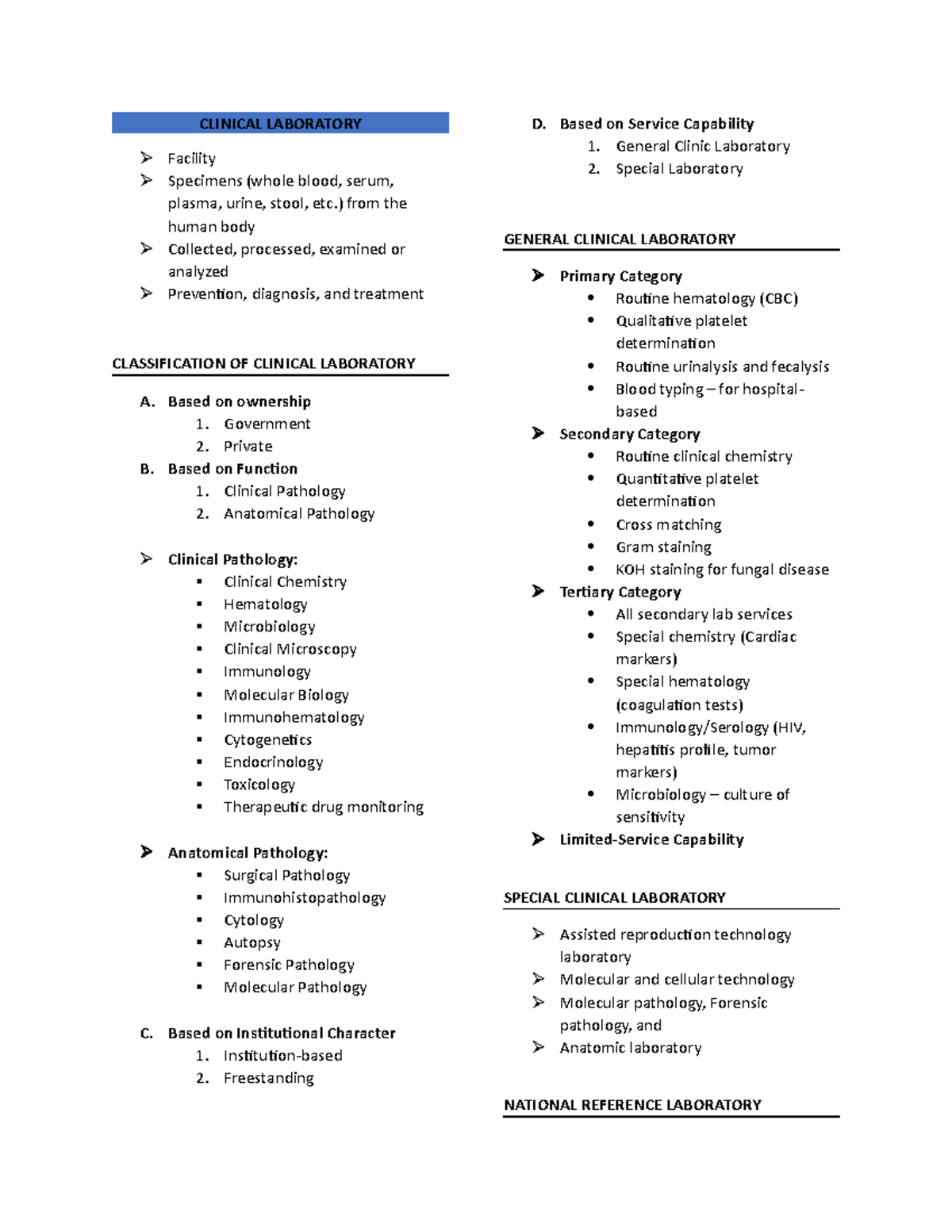This image displays a detailed categorization of clinical laboratory components and functions, arranged in two columns. At the top, a blue header prominently displays the title "Clinical Laboratory" in red letters. Below this header, several arrow-shaped bullet points list the types of specimens handled, including whole blood, serum, plasma, urine, stool, and other samples collected, processed, examined, or analyzed from the human body. These procedures support the prevention, diagnosis, and treatment of diseases.

A subsequent section features a new header, "Classification of Clinical Laboratory," underlined with a black line, and written in black letters on a white background. This classification is split into two main categories:

1. **Based on Ownership**:
    - Government
    - Private

2. **Based on Function**:
    - Clinical Pathology
    - Anatomical Pathology

Under the "Clinical Pathology" section, there are multiple key subfields, each highlighted by bullet points:
- Clinical Chemistry
- Hematology
- Microbiology
- Clinical Microscopy
- Immunology
- Molecular Biology
- Immunohematology
- Cytogenetics
- Endocrinology
- Toxicology
- Therapeutic Drug Monitoring

The visual layout emphasizes the comprehensive range of activities and specializations within a clinical laboratory setting.